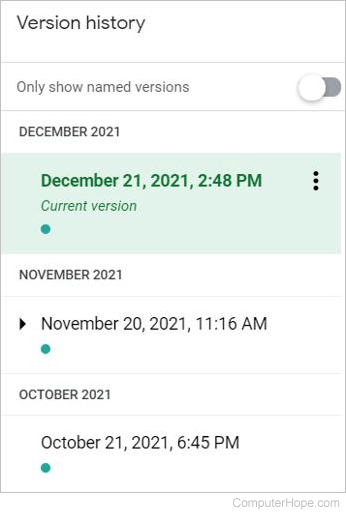A screenshot of a mobile device displaying the version history within a Google Doc. The interface has a white background with primarily black and grey text. At the top, the heading reads "Version history," followed by an option to "Only show named versions," which is currently toggled off. The visible history starts with "December 2021." The most recent version, highlighted with a slight green background, is dated "December 21, 2021, 2:48 PM." Following this, there is "November 2021," which can be expanded to show multiple entries, including one from "November 20, 2021, 11:16 AM," each marked with a green dot. Lastly, "October 2021" is shown, with a specific entry from "October 21, 2021, 6:45 PM," also marked by a green dot.